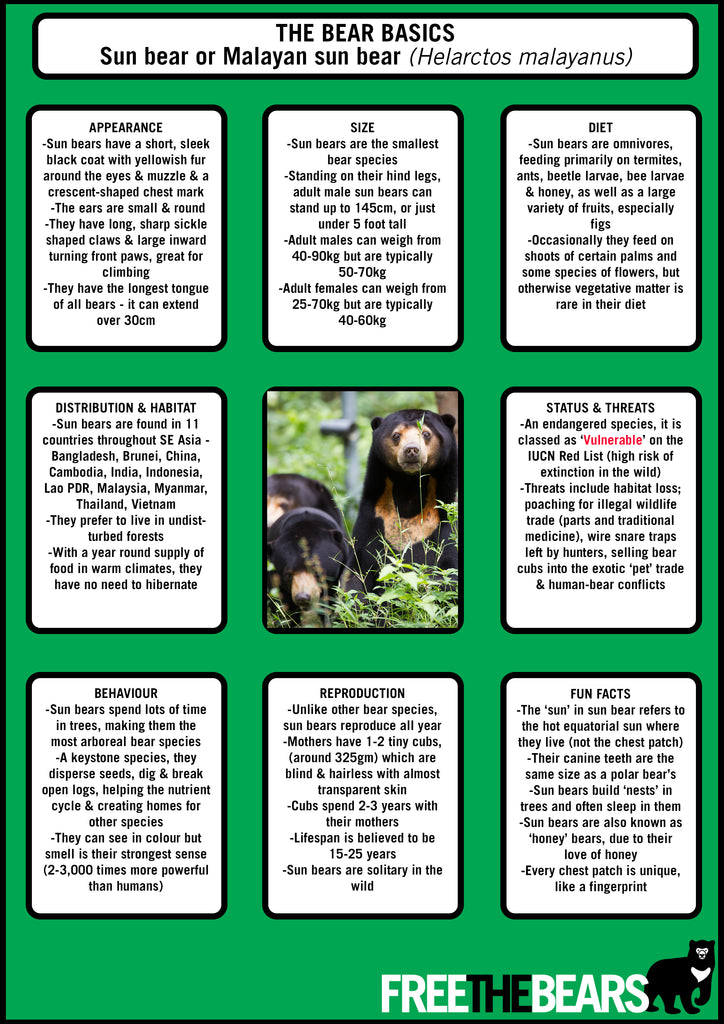The advertisement, titled "The Bear Basics: Sun Bear or Malayan Sun Bear (Helarctos malayanus)," provides a detailed overview of the sun bear. It features a green background with nine distinct, white-background, black-lettered sections, each bordered in black. Starting from the top left, the chart covers Appearance and then Distribution and Habitat. At the top center, information about Size is provided, followed by Diet in the top right corner. The middle row includes sections on Distribution and Habitat, a central photograph of three sun bears that are black with some brown on their face and chest, and Status and Threats. The bottom row is dedicated to Behavior, Reproduction, and Fun Facts. At the bottom right corner, a section labeled "Free the Bears" features a black and white drawing of a bear.